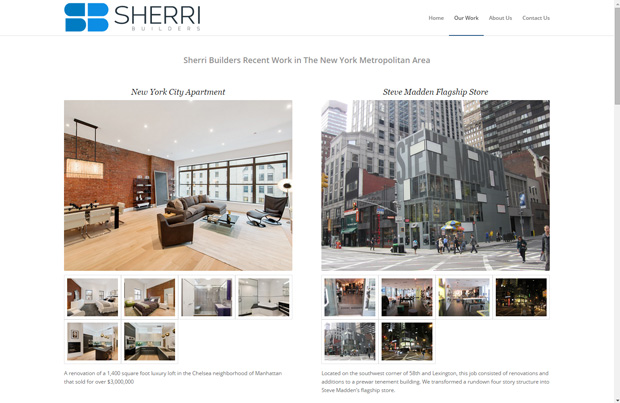A detailed caption for the image:

The screenshot is of a website called Sherry Builders. The logo is uniquely shaped like a tic-tac cut in half, with one half colored dark blue and the other light blue. To the left of the text "Sherry Builders," which is prominently displayed in larger lettering, there are two additional half tic-tacs in similar color combinations. On the right-hand side of the screen, a menu bar lists options including Home, Our Work, About Us, and Contact Us. The "Our Work" section is currently selected and underlined in blue.

Below the menu, there's a featured project titled "New York Apartment," showing a photograph of an apartment interior. The apartment features a brick wall, cozy furniture, a throw carpet, a kitchen table, and hanging lights. Underneath this image, there are additional photos showcasing various apartment interiors, including bedrooms, bathrooms, and kitchens.

Another project highlighted is "Steve Modern Flagship Store," which features an external image of the store located at the corner of 5th Street. The building is notable for its gray façade covered in what appears to be post-it notes obscuring the windows. Inside, the website offers a glimpse of the interior space, though the images are quite small and details are hard to discern. The site as a whole appears to focus on building and renovating projects, showcasing their portfolio of work in a highly visual manner.